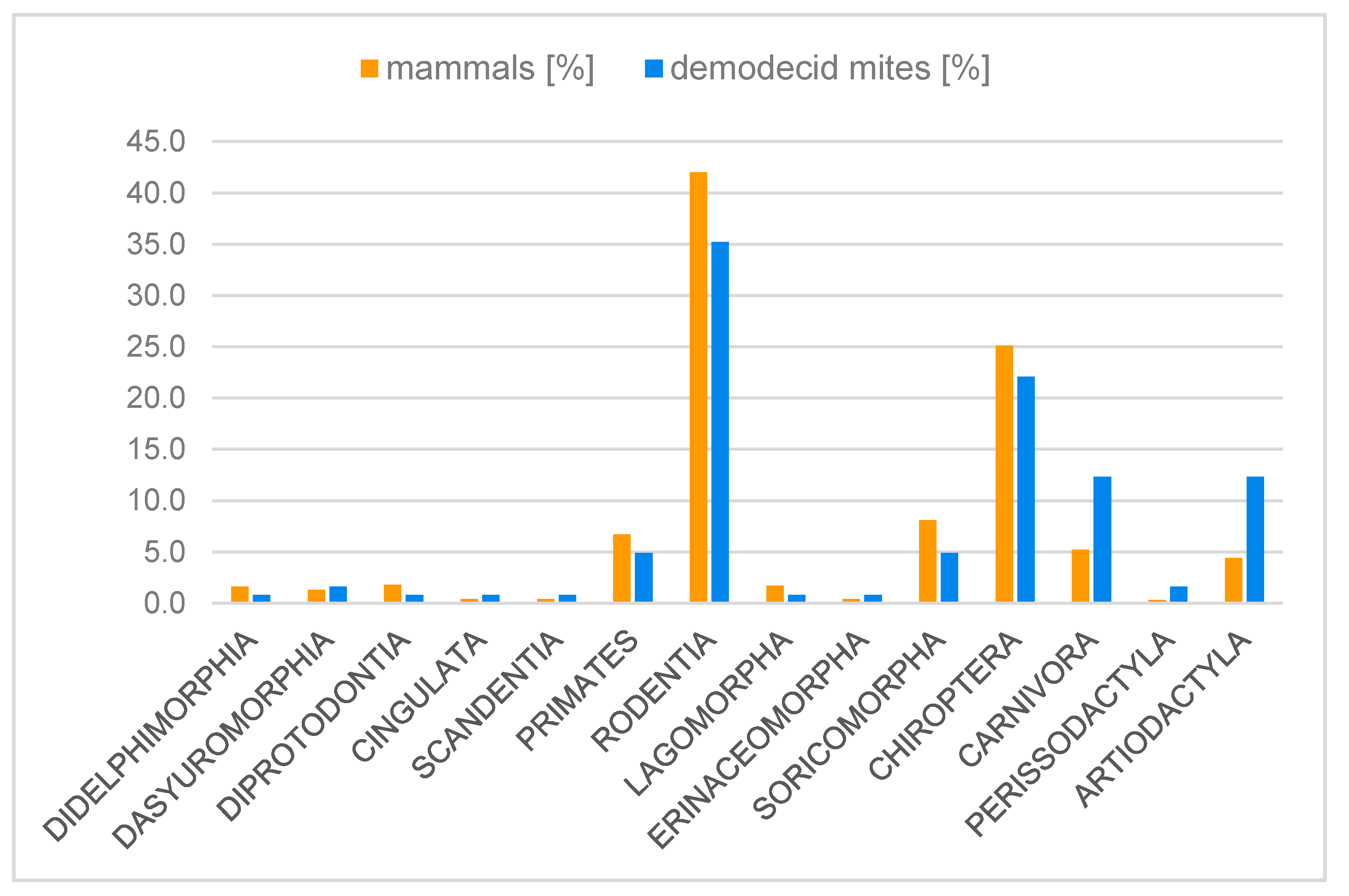The image features a detailed bar graph with various colors: white, black, light gray, orange, and blue. The bars are organized on a white background, measuring percentages on a vertical scale from 0 to 45 in increments of 5. At the top of the graph, there is a small orange square labeled "Mammals Percent" and a small blue square labeled "Demodecid Mites Percent." The x-axis categorizes several families or classes of animals, including groups such as Didelphimorphia, Primates, Rodentia, and Lagomorpha, totaling around 15 categories, each difficult to pronounce. Each category is paired with corresponding orange and blue bars, illustrating the percentage measures for both mammals and Demodecid mites. The entire graph occupies the full extent of the image, providing a clear comparative analysis of these percentages across different animal families.